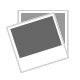This close-up product photo showcases a gold necklace meticulously arranged to display both its clasp and charm ends. The necklace, with its elegant gold chains, is artfully draped over a small wooden branch, creating a visually appealing contrast against the smooth, white microfiber surface beneath. Positioned on the left side of the image is the necklace's clasp, while on the right side, the charm, shaped like a pair of gold quotation marks, adds a unique touch. The overlapping chains form an X pattern in the center, enhancing the intricate presentation of this beautiful piece of jewelry.